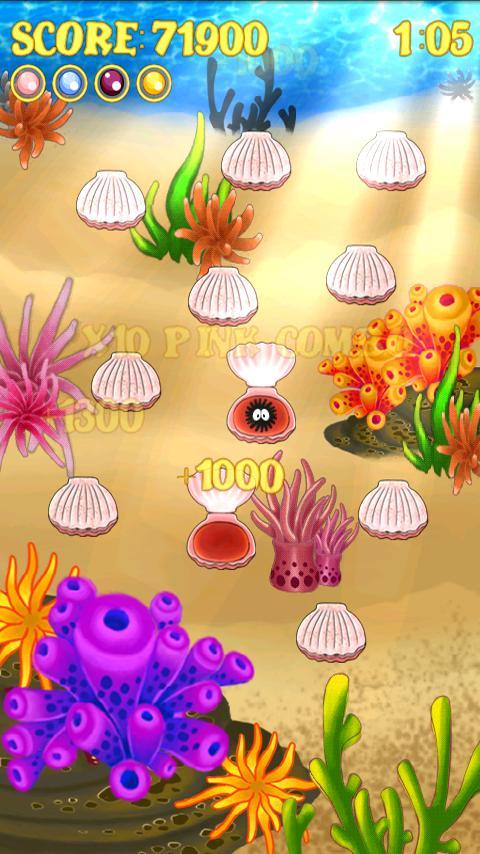The image depicts a vibrant, animated scene from a video game set in an underwater environment. At the top left corner, the score prominently reads 71,900, with a timer on the top right indicating 1:05 remaining. The central focus of the image is a collection of 11 clamshells arranged across a sandy ocean floor, with a shimmering blue water backdrop. Among the shells, two are open: one showcases a black, furry object resembling a spider, while the other is empty but marked with the number 1,000. Scattered across the scene, colorful coral reefs in hues of red, yellow, purple, pink, orange, and green add to the vibrant marine atmosphere. Below the score, multicolored circles with yellow rims—pink, blue, purple, and yellow—enhance the playful allure of this underwater-themed game.